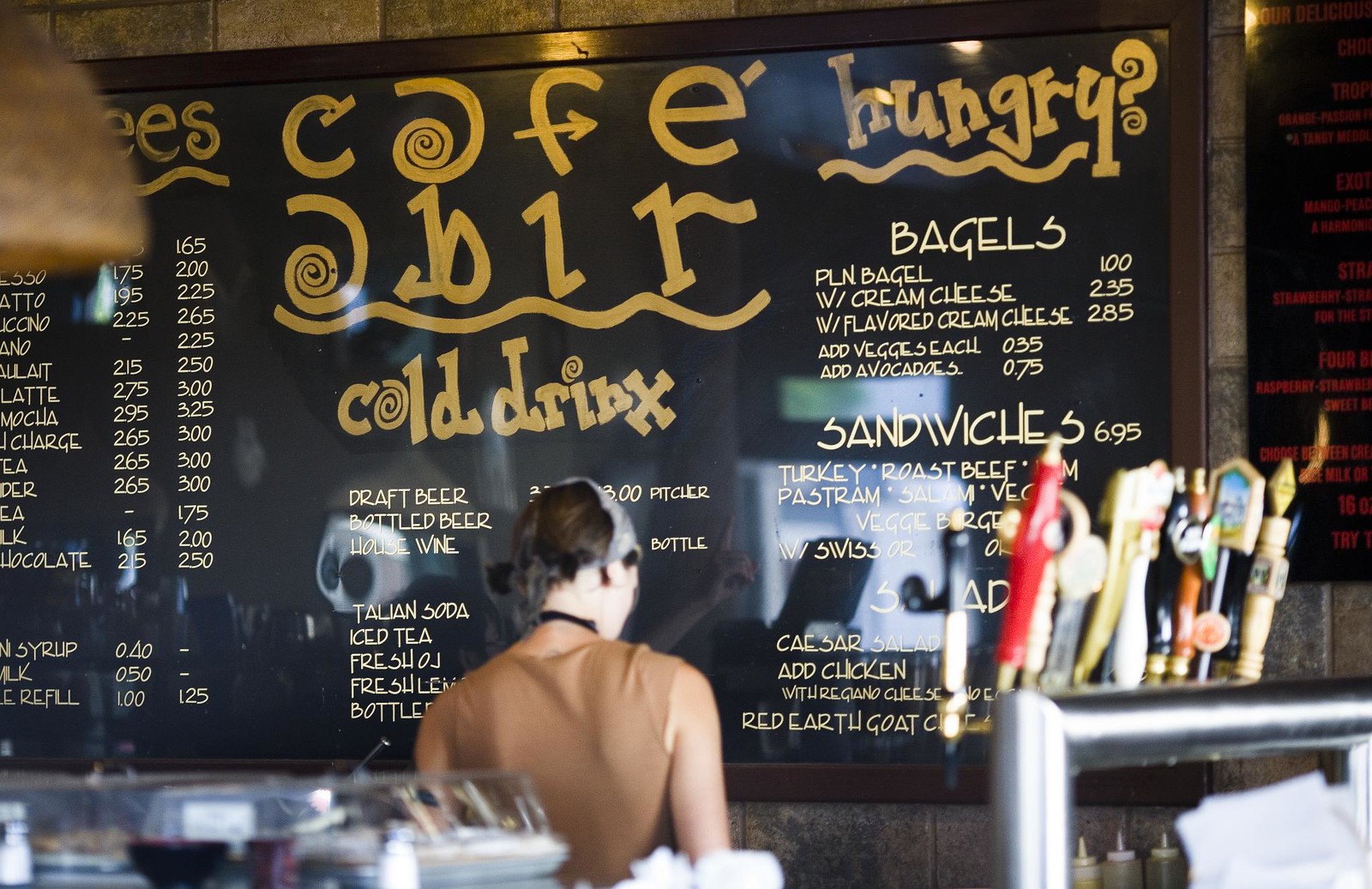In the image, a lady with her back to the camera stands in front of a large, framed blackboard menu affixed to a stone wall in a café. She has dark hair tied back with a gray handkerchief and is dressed in a sleeveless brown shirt, with a black strap around her neck. The menu prominently displays “Cafe de Beer” in yellow, stylized letters at the top, with an arrow through the "F" in "Cafe," and a decorative squiggly line beneath it. The menu is divided into sections: directly below the cafe's name, “Cold Drinks” are listed, including drafts, bottled beer, Italian soda, iced tea, and some items partially obscured. On the upper right, another section labeled “Hungry?” with a squiggly line and a question mark offers bagel options priced variably based on toppings like cream cheese and avocados, and also lists sandwiches such as turkey, roast beef, and pastrami. Below this menu section, there is an indistinguishable reflection obstructing some of the text, but "Writer’s Coat" can be discerned at the very bottom. To the right, a row of beer taps is visible, alongside some decorative pins standing atop a metallic bar. Behind the lady, additional café items like squeeze bottles, pastries, and containers can also be seen on the service counter.